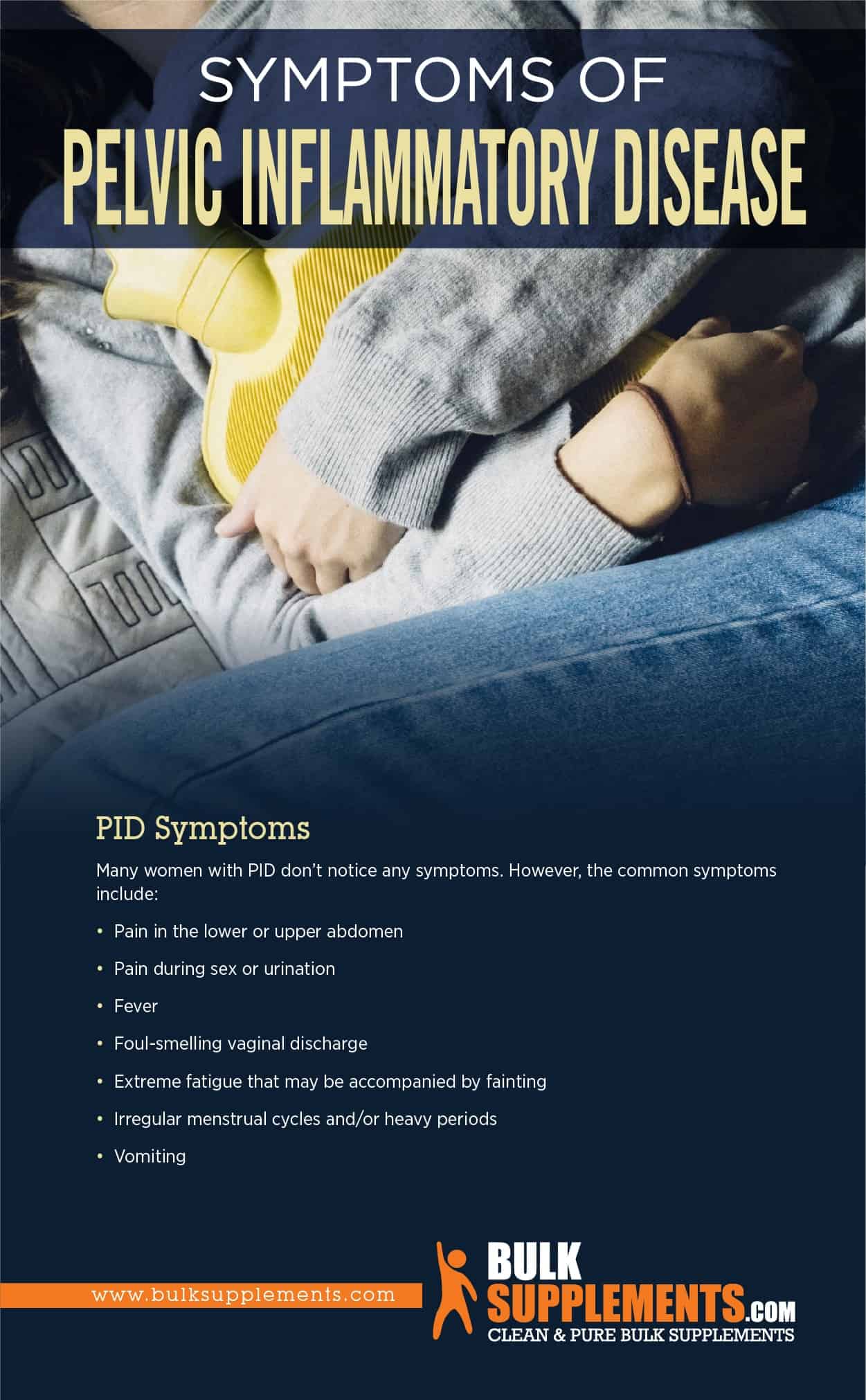The poster is an advertisement for BulkSupplements.com, promoting clean and pure bulk supplements. The background of the poster is blue, and at the top, it features the title "Symptoms of Pelvic Inflammatory Disease" in white and yellow text. The central image depicts a person curled up on a bed, with their arms wrapped around a yellow hot water bottle clutched against their torso. The individual, dressed in blue jeans and a gray sweatshirt, has one leg slightly pulled up diagonally across the image. A list beneath the image details common symptoms of Pelvic Inflammatory Disease (PID): pain in the lower or upper abdomen, pain during sex or urination, fever, foul-smelling vaginal discharge, extreme fatigue possibly accompanied by fainting, irregular menstrual cycles or heavy periods, and vomiting. The bottom of the poster features an orange bar with the URL "www.bulksupplements.com" and a logo of an outline of a human with one arm raised, along with the text "Clean and Pure Bulk Supplements."